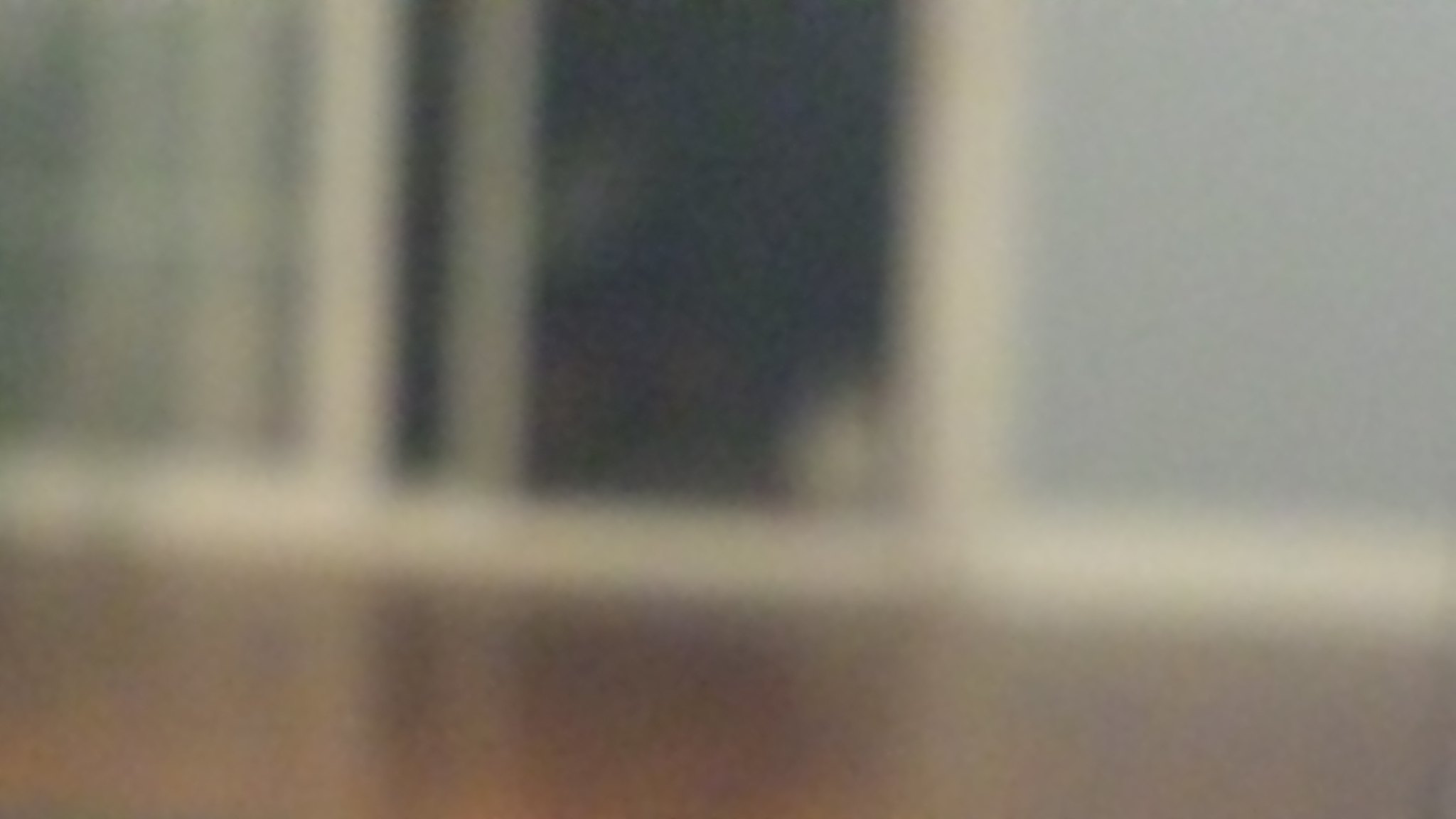The image depicts an extremely blurry scene featuring a seemingly interior setting. At the bottom of the frame, there's a brown wooden floor that transitions into a white floorboard, connecting the floor to the walls. Central to the image is a black doorframe, bordered by off-white or white wood. The surrounding walls display shades of gray—darker to the right of the door and a lighter shade or possibly a window to the left. Within the black doorway, there appears to be a faint light shape which is unidentifiable due to the blur. Just above this, light blue or white elements could suggest the presence of additional architectural features, potentially a window with black intersecting lines. Overall, the image primarily captures parts of a floor, door, wall, and potentially a window, all merging into an indistinct blur.